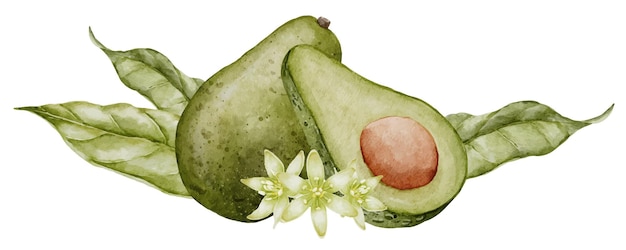The image depicts a detailed drawing of avocados on a white background. The composition includes one whole avocado and an adjacent half avocado revealing its large, pinkish-brown seed. The outer skin of the avocados is darker green, transitioning to a lighter green in the inner flesh. Behind the avocados, three two-toned green leaves with visible veins and thin, curly ends peek out. In front of the avocados, three small white flowers with faint green centers and stamens add a delicate touch. The avocados lean against each other, creating a balanced arrangement of the fruit, flowers, and leaves in the illustration.